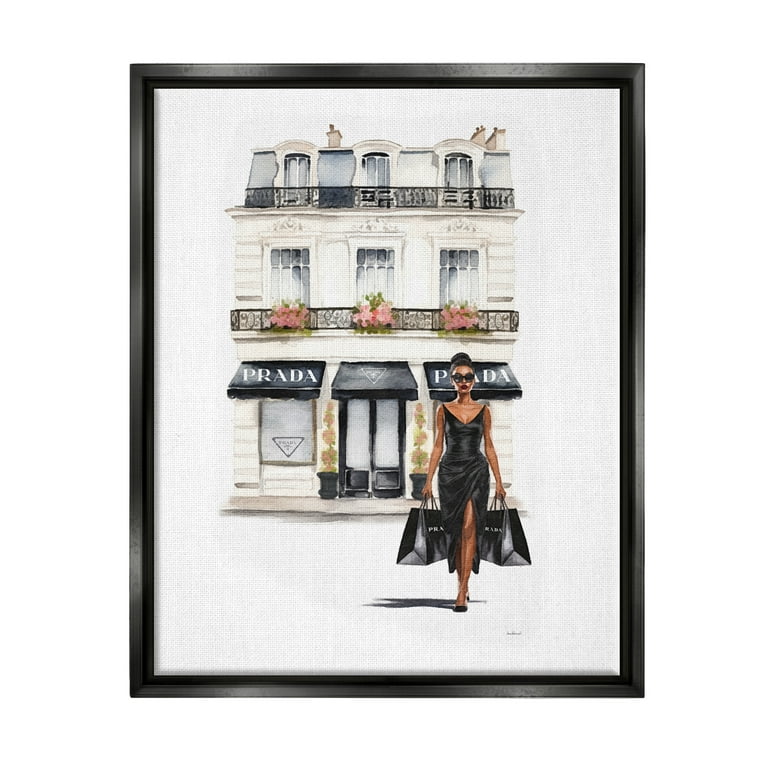The framed artwork, set against a white backdrop, showcases a detailed watercolor painting of a three-story, white building with ornate architectural features. The building, identifiable as a Prada store, has black awnings over the ground floor windows and doors, each bearing the white Prada logo in all caps. Above the awnings, the second and third stories each feature three windows, adorned with balconies overflowing with pink flowers, adding a touch of vibrancy to the scene.

In the foreground, a sophisticated woman is depicted walking towards the viewer. She is dressed in a chic black evening gown with a thigh-high slit on her left side, complemented by high heels. Her black hair is neatly styled in a bun atop her head, and she wears dark sunglasses and striking red lipstick. The woman carries two black garment bags, likely containing her recent purchases from the store, which subtly display the Prada logo. The entire scene is captured within a sleek black frame, creating a stylish and elegant presentation.